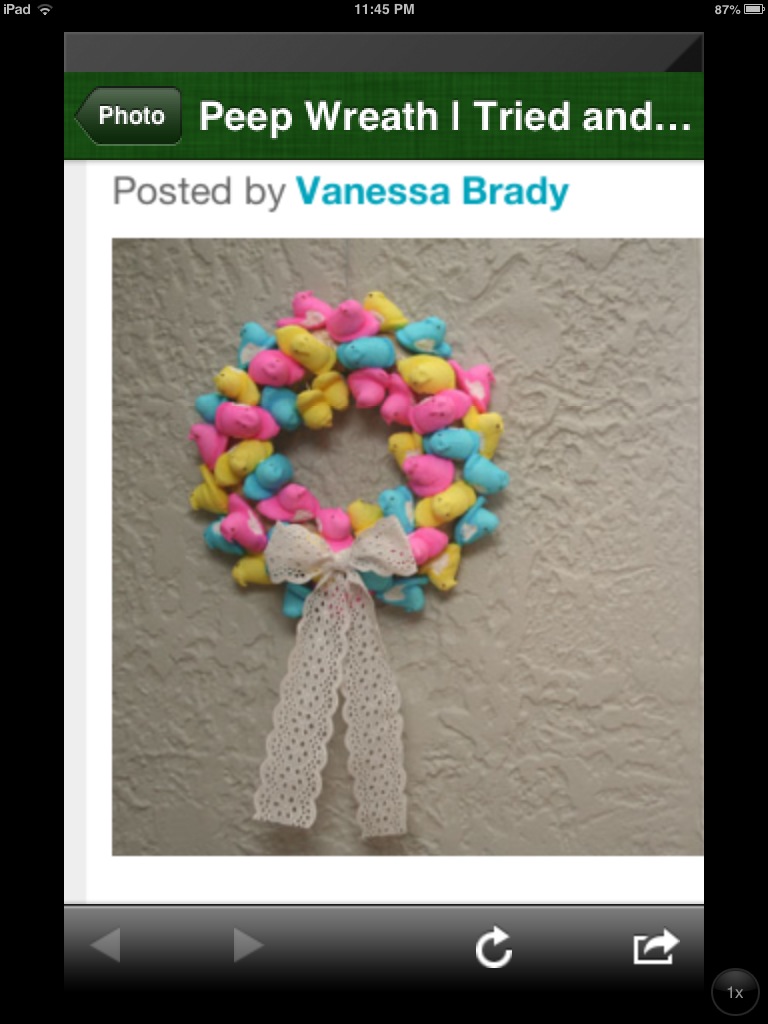This image is a screenshot of an iPad displaying a screenshot from an iOS device photo viewer. The iPad UI shows it is 11:45 p.m., with a Wi-Fi connection and 87% battery remaining. The main focus is an image of a wreath made entirely of pink, yellow, and turquoise marshmallow peeps. The wreath is tied at the bottom with an ivory-colored lace bow and is displayed against a light gray stucco wall. The borders of the image are white and black, set on an ivory-colored textured background. Text overlaying the image reads "peep wreath I tried and..." followed by "posted by Vanessa Brady" with "Vanessa Brady" in turquoise and "posted by" in gray. The viewing UI includes standard photo navigation and action buttons at the top and bottom.